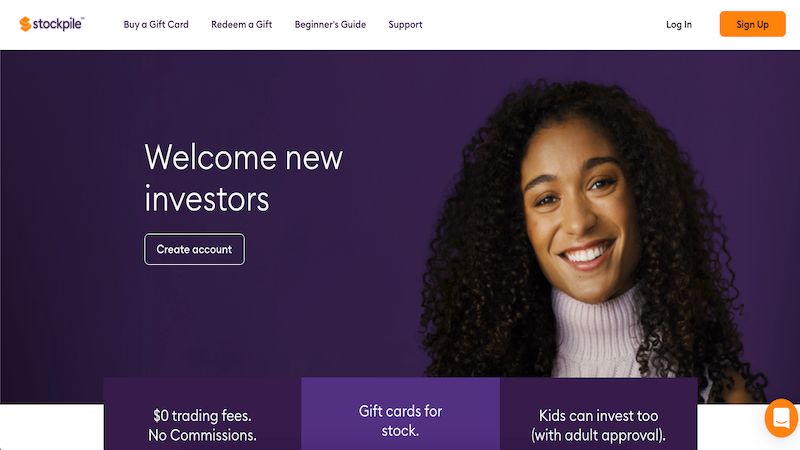The Stockpile website features a clean and welcoming layout designed for new investors. At the top left, the Stockpile logo is displayed, with "Stockpile" written in purple font and a distinctive orange "S" serving as the logo. 

To the right of the logo is a navigation menu that includes options such as "Buy Gift Card," "Redeem a Gift," "Beginner's Guide," and "Support." Further to the right on the same bar are the "Login" and "Sign Up" buttons for easy account access.

Beneath the navigation bar is a prominent, horizontally-oriented banner. The banner features a gradient effect, transitioning from a darker purple on the left to a lighter purple on the right. Positioned towards the left-center of the banner is the welcoming message, "Welcome New Investors," written in white font. Directly below this text is a white-outlined button with "Create Account" inscribed in white font, inviting users to get started.

The right side of the banner showcases a close-up image of a woman with black hair, smiling warmly at the camera, contributing to the welcoming and friendly atmosphere of the website.